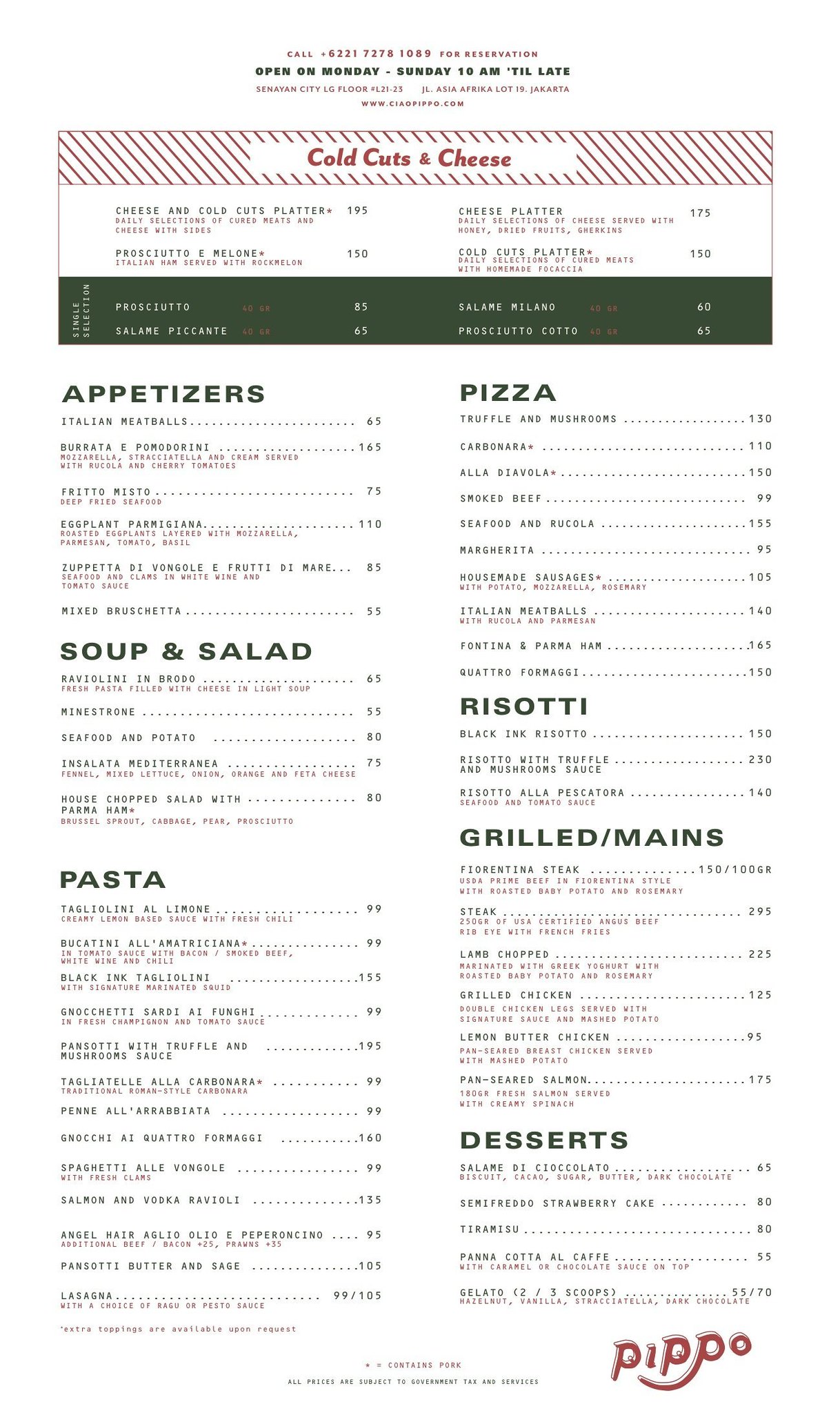The image presents a detailed menu for an Italian restaurant named Pippo, characterized by a white background and accented with green banners and some red text. At the top eighth of the menu, there is a section for cold cuts and cheeses highlighted in a red stripe, listing items such as prosciutto, salami picante, Milano, and prosciutto cotto, with prices like cheese and cold cut platter for $1.95, and cheese platter for $1.75. The menu is composed mainly of black text with various sections organized into columns: on the left, it lists appetizers, soup and salad, and pasta, while on the right, it details pizza, risotti, grilled mains, and desserts. The name "Pippo" is prominently displayed in the bottom right corner, written in fun pink letters. This organized layout and the traditional Italian offerings suggest an inviting Italian dining experience.